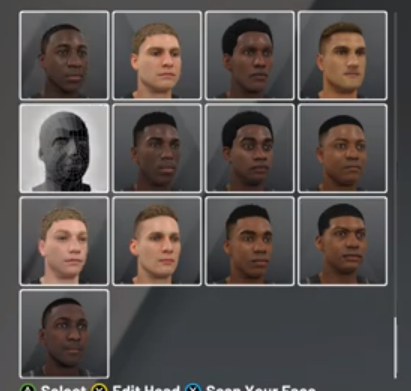The image is a detailed screenshot from a video game's character selection screen. It features a layout of 13 computer-generated profile images of potential player avatars, arranged in a grid formation. These avatars are diverse, consisting of men from different races with some characters being black while others are white. The grid is organized into four rows, with the last row containing a single profile image. 

In the second row, the first box contains a 3D rendering that appears to be an early-stage model of a character's head. This incomplete rendering is set against a grey background, showing the character's head still in the construction phase, without any skin or final textures applied. Each profile image is neatly bordered with a white outline, reinforcing their selection capability. The overall design suggests these characters are intended for a sports-themed video game, and the player is to choose one of these avatars to play as.